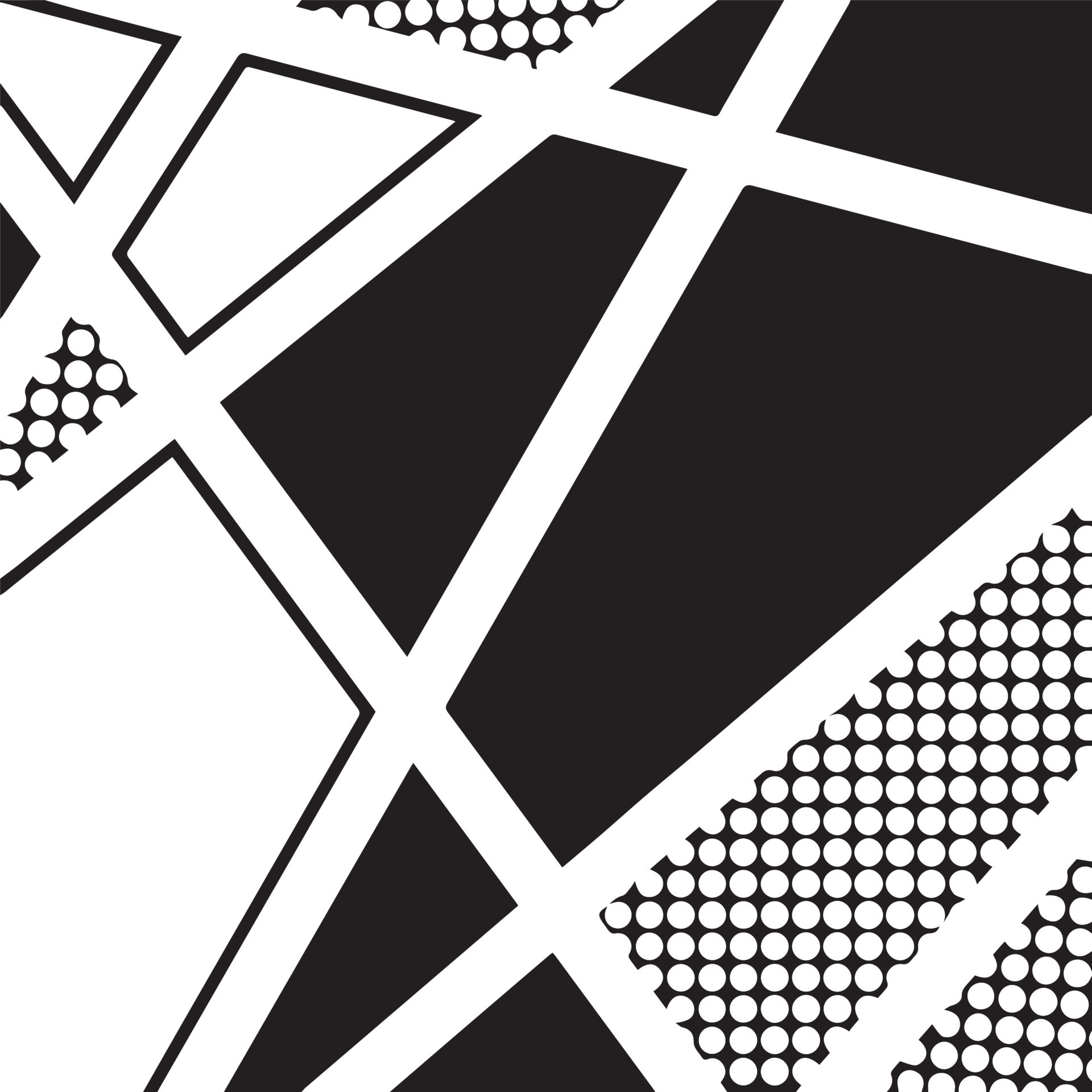The image depicts an intricate black and white abstract artwork characterized by a web of intersecting lines and irregular geometric shapes. Dominated by randomly angled diagonals, the lines create a dynamic network that fragments the canvas into unique sections. These sections vary greatly in shape, including near-triangular, trapezoidal, and irregular five-sided forms, none of which are identical. Certain intersections are filled in solid black, while others are solid white or feature black backgrounds with white polka dots. The white lines, about a quarter inch thick, weave through the artwork, enhancing the bordered effect and contributing to the appearance of a road map converging and diverging at various points. Notably, the middle section includes five distinct black parts, and additional black elements are scattered throughout, including a tiny triangle at the top left edge and two circular patterns near the bottom right. This composition, devoid of text or attribution, captivates with its diverse and meticulously organized abstract patterns.